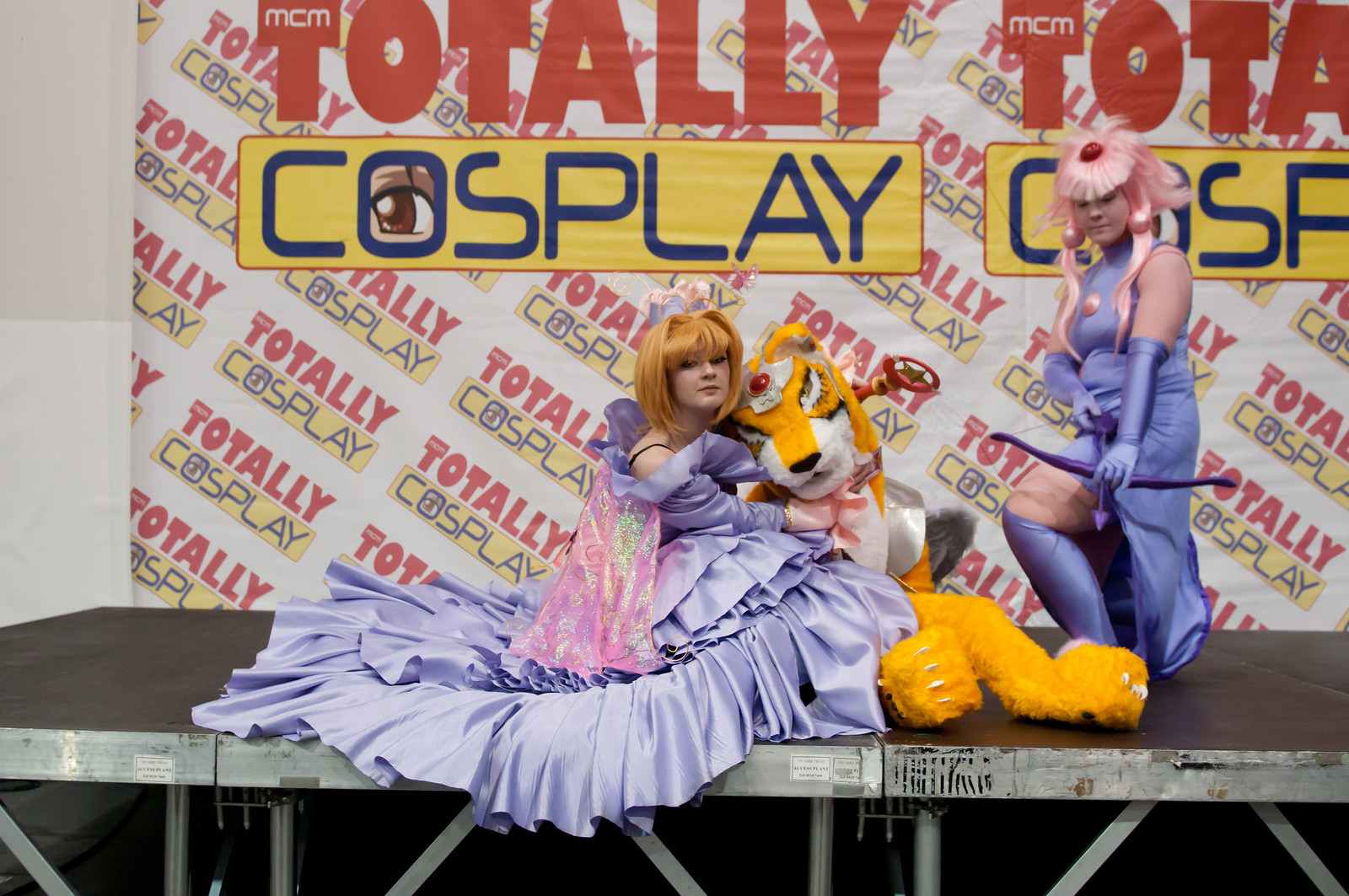The image captures a vibrant scene at what appears to be a comic convention, specifically on a stage with a black platform and steel frame, illuminated by bright lights. Dominating the backdrop is a large, eye-catching display that reads "Totally Cosplay" in a yellow border with blue font, interspersed diagonally in a grid pattern, each "o" featuring a human eye graphic.

On the stage, there are two young women, likely cosplaying as characters from Japanese anime. The girl on the left is seated, her long, flowing purple satin dress adorned with a pink, glittery cape, cascading over the stage floor. She has striking orange hair with large bangs and white skin. Next to her, she holds a large stuffed tiger with a metal helmet and a jewel on its forehead. 

The girl on the right, standing or slightly lunging, features an elaborate outfit as well. She sports vibrant pink hair styled with large pink balls, large bangs, and two locks hanging down the front. Her attire consists of a form-fitting, purple satin dress with matching long gloves and knee-high stockings. She accessorizes with purple earrings and a red cylindrical headpiece, and holds a purple bow and arrow, her eyes closed and head slightly bowed.

In the background, the stage is complemented by white walls, adding contrast to the colorful scene unfolding in front.